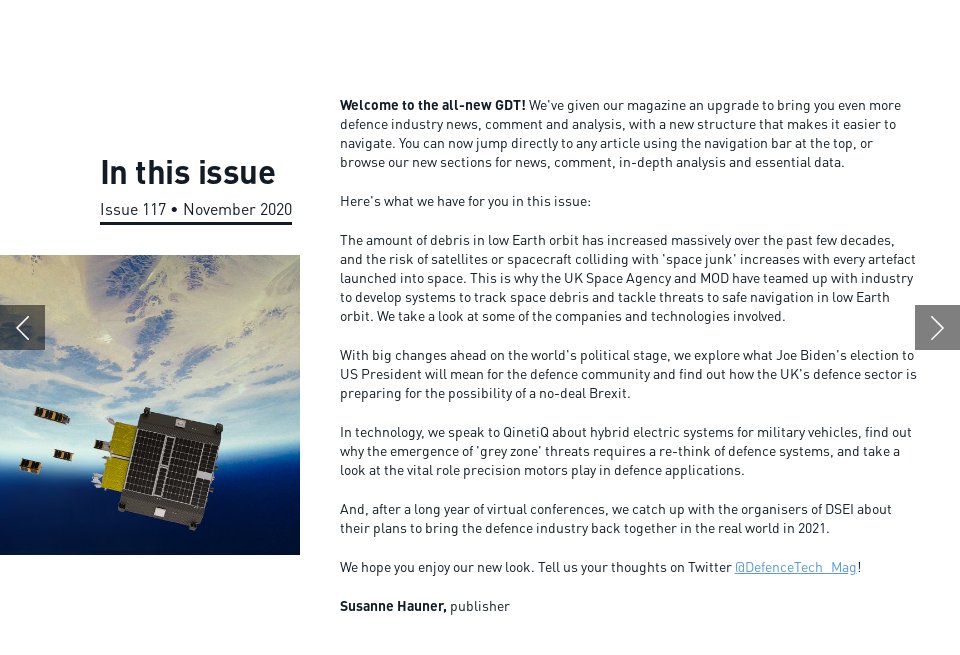The webpage features an article set against a white background with a prominent image on the left-hand side. The image appears to be a photograph captured from space, showing Earth from afar. The Earth’s surface, adorned with blue hues and cloud formations, is visible in the background. In the foreground of the image are five satellites. The closest satellite to the viewer is a significant, square-shaped object, equipped with solar panels on its top and adorned with golden-colored boxes on its sides.

Above the image, black text reads: "In this issue, Issue 117, November 2020," with the issue number and date underlined for emphasis. To the right of the image lies the introductory text of the article.

The article announces the introduction of the newly upgraded "GDT" magazine, aimed at delivering enhanced defense industry news, commentaries, and analyses. The new format promises easier navigation and the ability to jump directly to any article through a navigation bar at the top. The magazine now includes new sections dedicated to news, commentaries, in-depth analyses, and essential data.

The specific topics covered in Issue 117 include the rising amount of debris in low Earth orbit and the subsequent collision risks posed to satellites and spacecraft. It discusses the collaborative efforts between the UK Space Agency and the Ministry of Defence (MOD) in developing tracking systems to handle these threats.

The article also delves into the implications of Joe Biden's presidential election for the defense community and explores how the UK's defense sector is preparing for a potential no-deal Brexit. 

In the technology section, there are discussions with KinetiQ about hybrid electric systems for military vehicles, an examination of the emerging "gray zone" threats and their impact on defense strategies, and insights into the critical role of precision motors in defense applications.

Closing the article is a feature on DSEI organizers, who share plans for resuming in-person defense industry gatherings in 2021 after a year dominated by virtual conferences.

The article concludes with an invitation for readers to share their feedback on Twitter at @defensetech_mag, and the publisher, Suzanne Hauner, signs off with her name boldly emphasized.